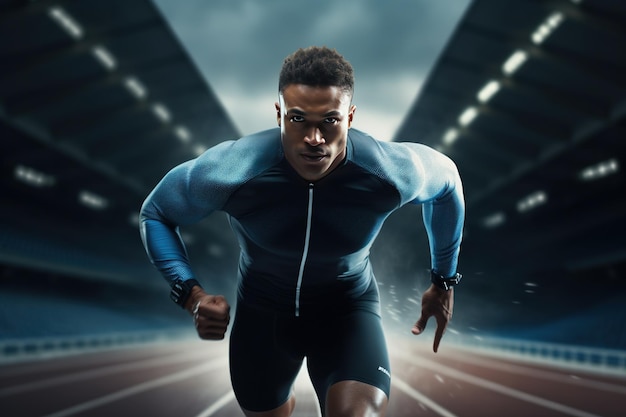In the foreground of the image, a black man with short, curly hair is sprinting towards the viewer on a racetrack. He is clad in a blue tracksuit, with a darker blue shade on his chest and shorts, and a lighter blue on his sleeves. The outfit features a visible zipper down the front. On both wrists, he appears to be wearing oversized watch-like objects. The background consists of an empty stadium with white fences lining the track, and stands that are blue, suggesting seating areas for spectators. The sky overhead is cloudy with a hazy appearance. This image gives off a futuristic, AI-generated feel, with noticeable artifacting and some proportional anomalies, particularly in the man’s oversized upper body and hands.